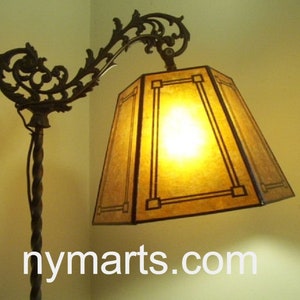The image showcases an intricate floor lamp labeled with the website "NYMARTS.com" in white text at the bottom. Positioned against a golden-yellow or tan wall, this metal lamp, possibly in dark brown or black, is a key focus. The base of the lamp features detailed vine or scroll-like decorations that extend upwards. The lampshade, reminiscent of a six-sided lantern, is constructed from glass panes forming sloped rectangles bound by black borders, with more intricate rectangular designs inside, formed by interconnected rods and squares. The shade is topped with parchment-like paper in a darker goldish-brown hue, allowing the bright, glowing light to shine through and illuminate the scene. The power cord discreetly winds down the lamp, blending into its ornate structure.